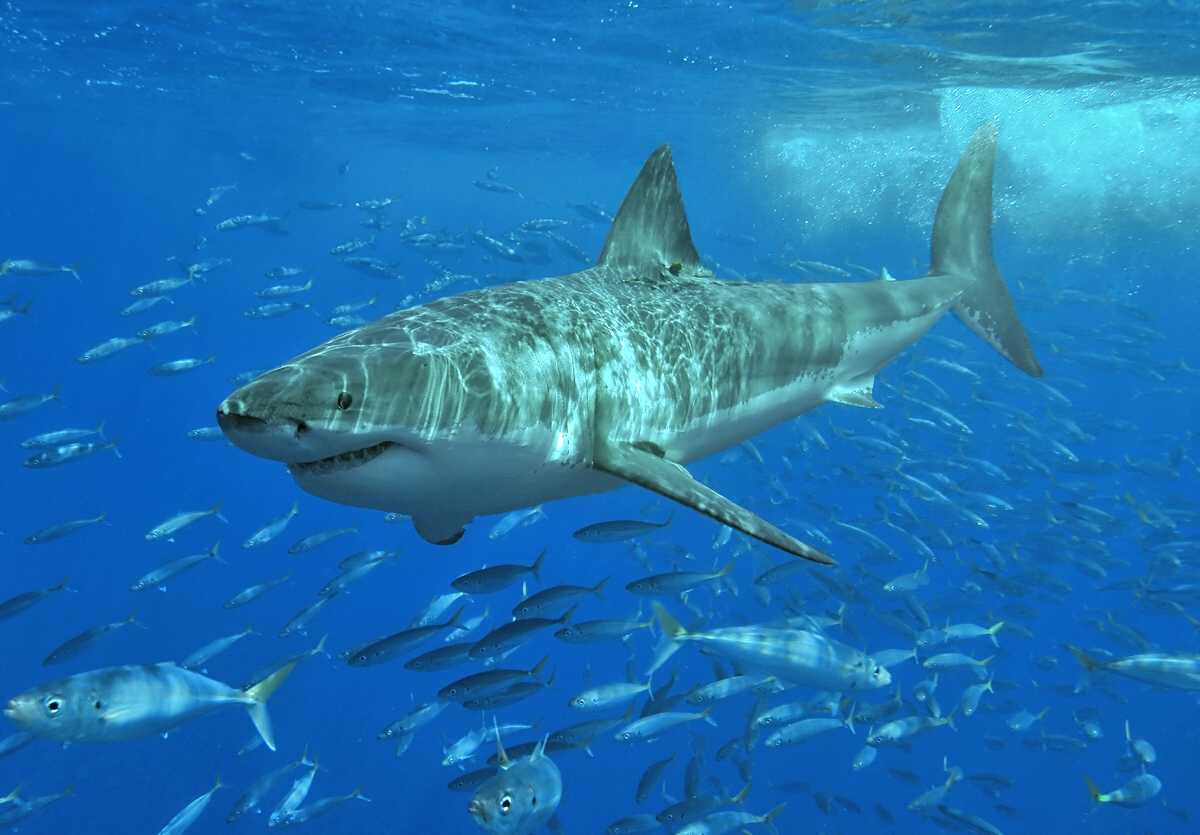The image captures an underwater scene dominated by a massive shark, likely a great white, exhibiting the typical coloration of green on top and white underneath. The menacing teeth and singular visible eye are prominent features as it swims powerfully through the deep blue sea. Surrounding the shark is a vast school of small fish, numbering in the hundreds, varying in hues from blue to green-tinged tails. These fish, some appearing to have horn-like appendages, scatter around the shark, which seems to be on the prowl, potentially searching for its next meal. The water is penetrated by streaming lines of light, illuminating the shark's snout and the dynamic motion of its tail, which creates a trail of bubbles, further emphasizing the sense of movement in this vibrant, aquatic tableau.